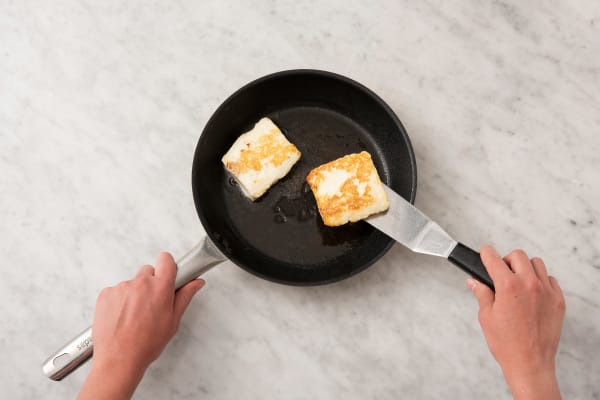In the image, we see a top-down view of a cooking scene on a grayish-white marble countertop. A pair of white hands are shown in the midst of preparing a dish. One hand holds a medium-sized, black skillet with a silver handle, while the other manipulates a metal cake spatula with a black handle. The spatula lifts a piece of bread that is square-shaped and toasted to a golden brown, possibly having been fried in butter or oil. The bread on the spatula and in the skillet has hints of orange, suggesting a topping of browned butter or melted cheese. The pan appears to be Teflon coated, and the well-lit kitchen environment accentuates the tiny details of cooking in progress.